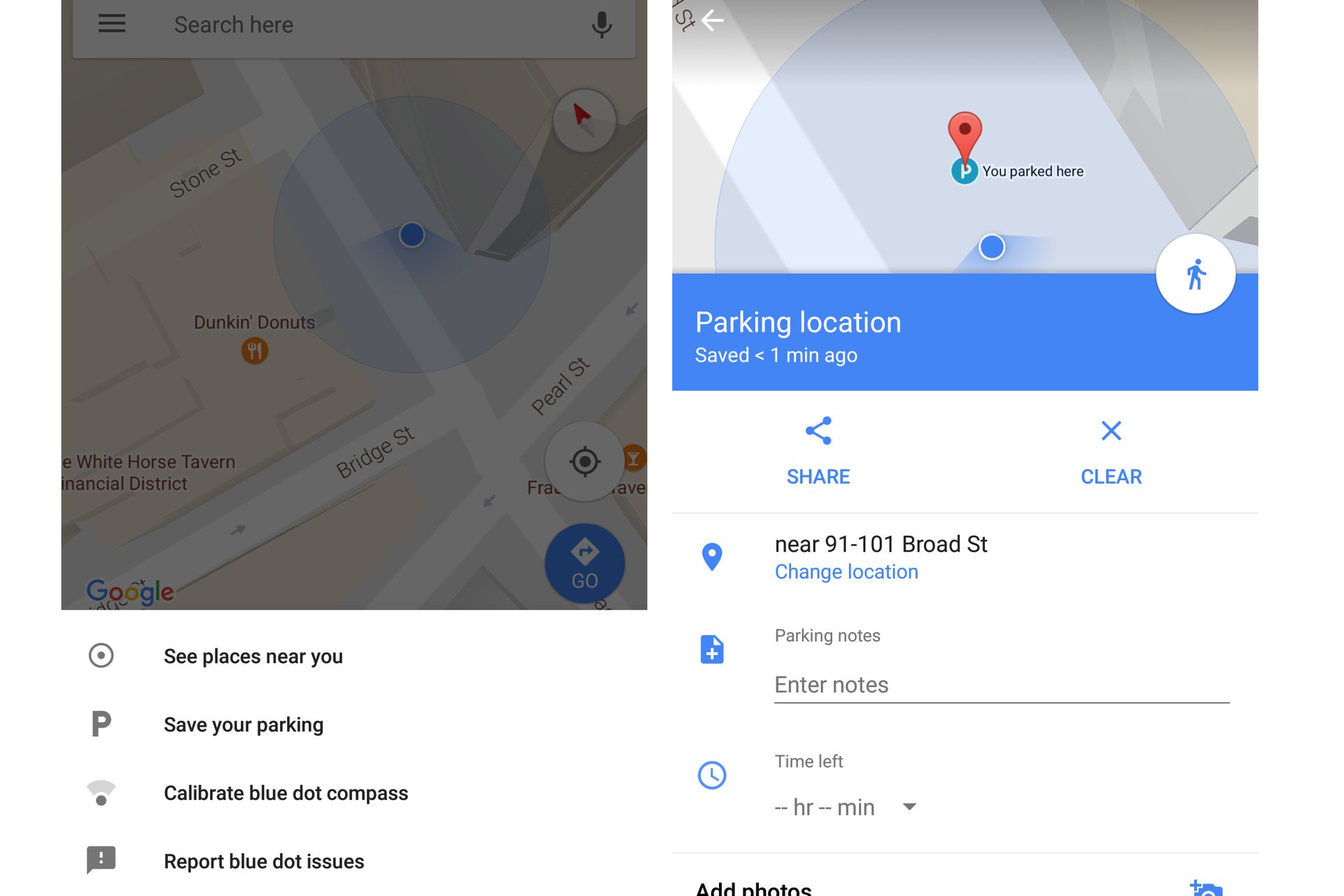The image showcases two distinct map interfaces side by side, each filled with intricate details.

**Left Map:**
- The map prominently features a blue dot indicating a user's location, surrounded by a blue radius.
- Streets visible on the map include Pearl Street, Bridge Street, and Stone Street.
- Notable landmark: Dunkin' Donuts.
- A compass is displayed for orientation purposes.
- At the top of the map, there's a search box labeled "Search here" accompanied by three horizontal lines representing settings and a microphone icon for voice input.
- Below the map, options are listed to "See places near you," "Save your parking," "Collaborate," "Calibrate blue dot compass," and a gray box with a caution sign that says "Report blue dot issues."

**Right Map:**
- The map highlights a red location marker indicating "You parked here," alongside the blue location dot.
- A notation below reads "Parking location saved one minute ago," with options to "Share" and "Clear."
- Displays address: "Near 91-101 Broad Street," with an option to "Change location."
- A section for "Parking notes" with an "Enter notes" field.
- A "Time left" function to presumably monitor parking duration.
- Design elements include a clean, white background with black text and blue links, maintaining readability.
- Additional icon: A button depicting a walking figure, useful for navigation or pedestrian routes.

Overall, the design is functional and user-friendly, with necessary navigation and location features prominently displayed against a minimalist interface.